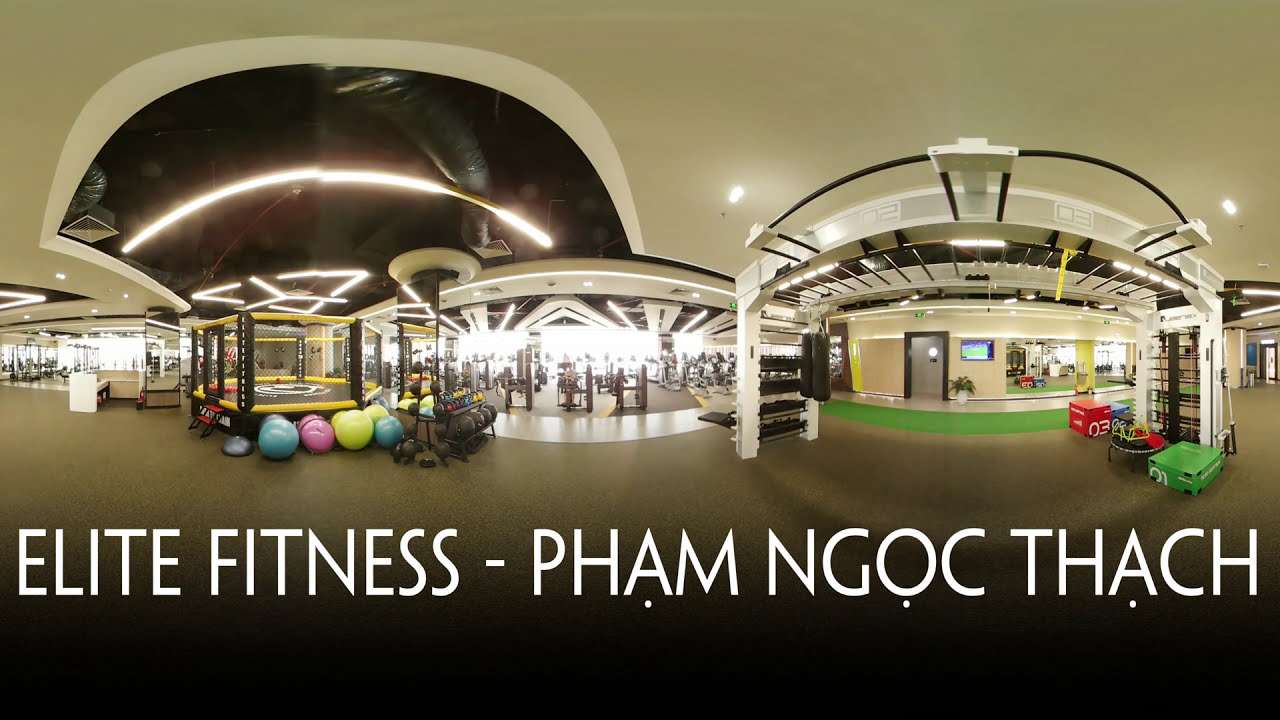The image showcases a spacious and sophisticated gym named "Elite Fitness Pham Tham Ngoc Thach," prominently labeled in large, strong white letters across the bottom. The gym features an impressive design with beveled archways, including three in the background and a main archway leading to the entrance, which is well-illuminated and reveals a variety of weight machines. The floor is covered with a green, fuzzy carpet that traverses the gym. In front of the far archway, there's a distinctive black and yellow trampoline-like object with a net enclosure, surrounded by various colored fitness balls in turquoise, pink, and fluorescent green. To the right, an octagonal sparring arena is visible, contributing to the gym’s diverse equipment, which also includes weight training areas. The gym exudes a clean, organized, and professional atmosphere, appealing to fitness enthusiasts.